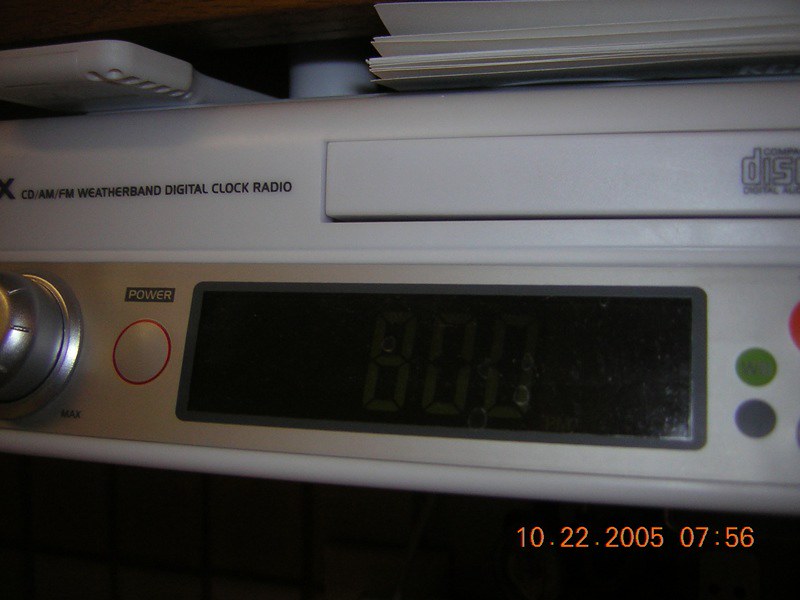In the bottom right corner, the image is marked with the timestamp "1022.2005, space 07, 56." In the top left quadrant, there's a first view of a CD player integrated with AM, FM, and weather band radio, alongside a digital clock display. To the immediate right, a rectangular label reads "Compact Disc Digital Audio." Also in the top left section, there’s a piece of white plastic. In the top right, there’s a stack of papers. 

In the bottom left corner of the image, a silver die can be seen. Just to its right is a black rectangle marked with "Power Up" and a white button followed by a red circle. The digital display located in the center is unlit, showing a black screen. The middle part of the display faintly indicates the number "800," designed using segmented digital lights. To the right of this display, a small circular green button labeled "WB" is visible, along with a blue button next to it. There is also a hint of red, slightly off-screen, on the right-hand side.